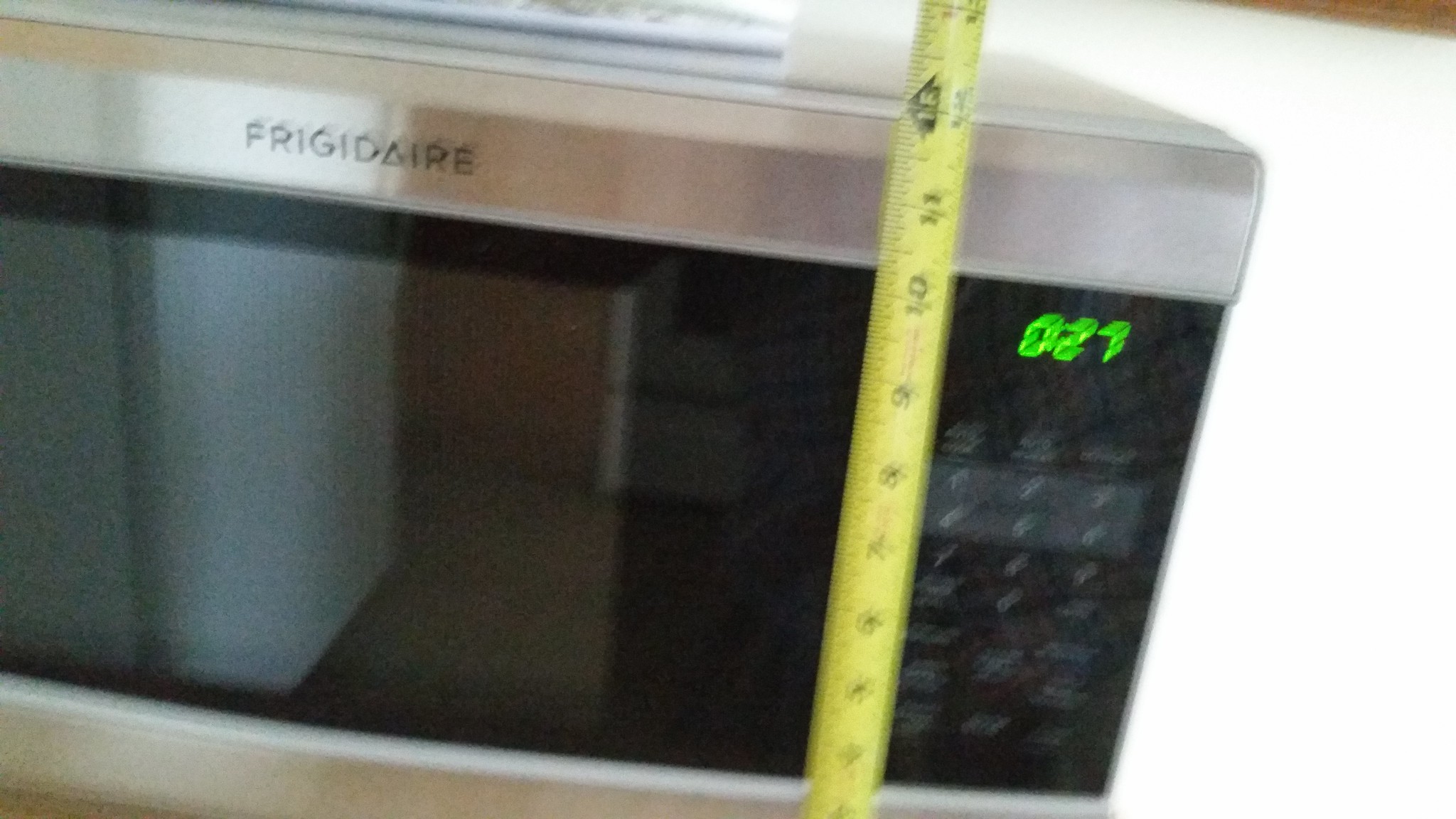The photograph is a blurry, out-of-focus close-up of a Frigidaire microwave. The microwave, adorned with the Frigidaire brand name at the top center, features a sleek design with metallic silver finishes on the top and bottom and a black door and control panel. The control panel, situated on the right, includes white-lettered buttons and an LED display currently showing "0:27." A yellow retractable measuring tape stands upright in front of the microwave, indicating its height to be precisely 12 inches, or one foot. Despite the poor image quality and the off-kilter angle, the photograph captures the essential details, including the microwave's color scheme and the measurement context. In the background, a white table or counter is partially visible.